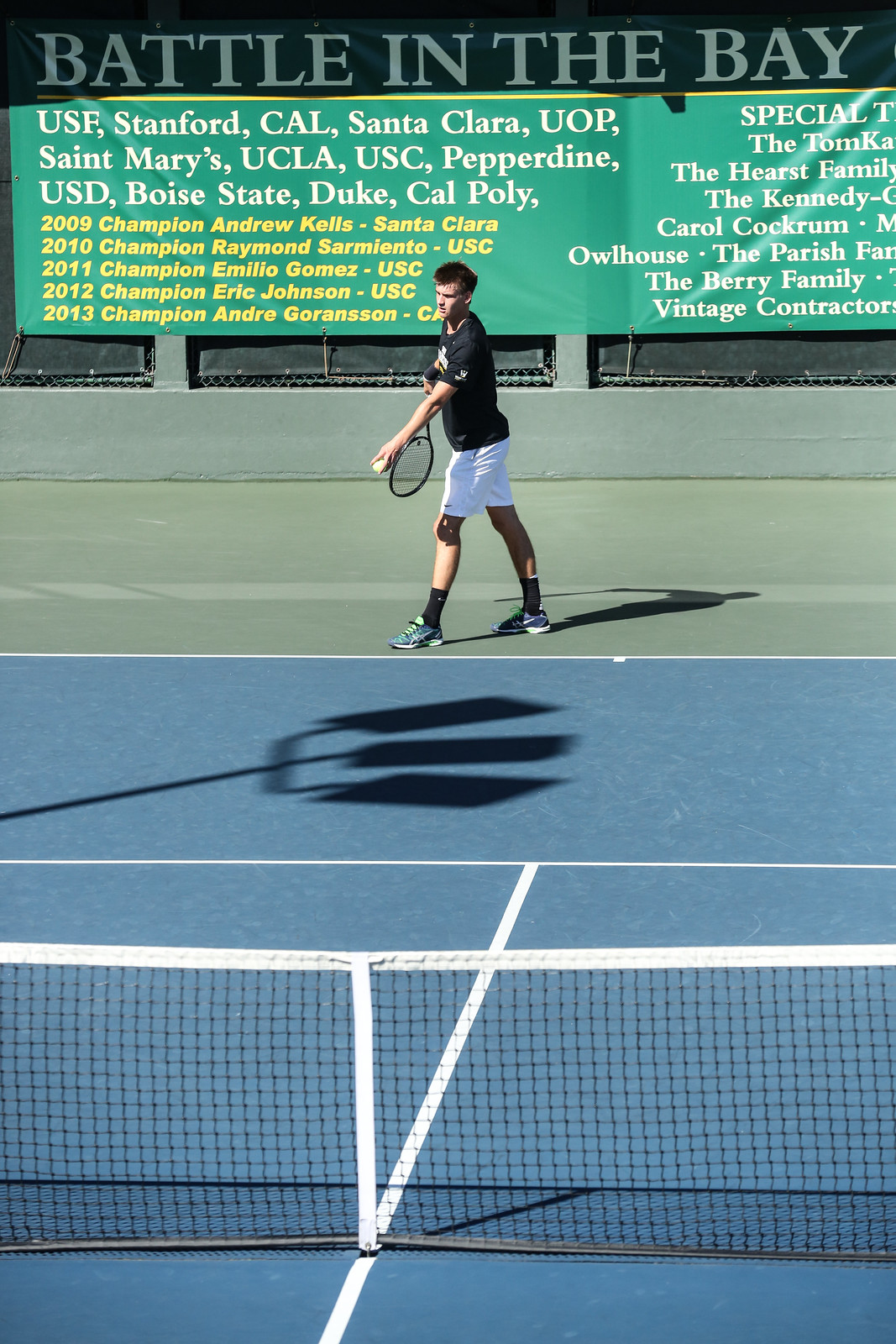The photograph captures a bright, sunny day at an outdoor tennis court, vividly blue with crisp white stripes. Right in front of you stands a white net, and on the far side of the net is a young, dark-haired Caucasian man preparing to serve. He is dressed in white shorts, black socks, a black t-shirt, and tennis shoes, holding a tennis ball in one hand and a tennis racket in the other. Behind him stretches a large green banner emblazoned with "BATTLE IN THE BAY" in white, all-caps lettering at the top. Below this, in white letters, are the names of several universities: USF, Stanford, California, Santa Clara, UOP, St. Mary's, UCLA, USC, Pepperdine, USD, Boise State, Duke, and Cal Poly. Beneath these, in yellow, the banner lists champions from 2009 to 2013 – Andrew Kellis (Santa Clara), Raymond Ceremento (USC), Emilio Gomez (USC), Eric Johnson (USC), and Andrea Gordonson, though the rest is cut off. On the right side of the banner, additional print is visible but not completely legible. The scene conveys a moment of intense concentration as the player prepares for his serve, framed by the accolades and history of the surrounding collegiate tennis competition.